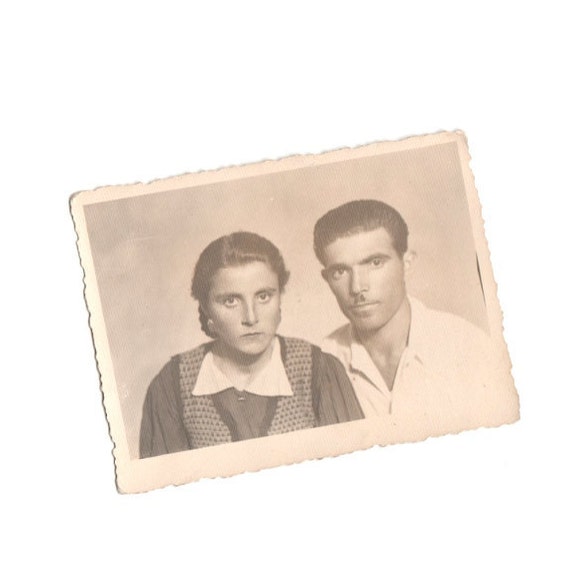This is a vintage photograph that appears to be from the 1920s to 1950s, featuring a young couple dressed in period clothing. The image itself is monochromatic with a sepia tone, giving it an aged appearance, and the edges of the photo are frayed, enhancing its vintage look. 

The woman, positioned on the left, has dark hair and wears a patterned sweater vest over a dark-colored shirt with a collar. She gazes directly at the camera with a serious expression. The man, on the right, has black hair and a small mustache reminiscent of a "Hitler stache." He wears a light-colored shirt and looks away from the camera. Both individuals stand in front of a plain wall background, their expressions neutral as if this image was one of many taken during a photo session. The overall tone of the photograph is light tan, indicating its age and giving it a nostalgic feel.